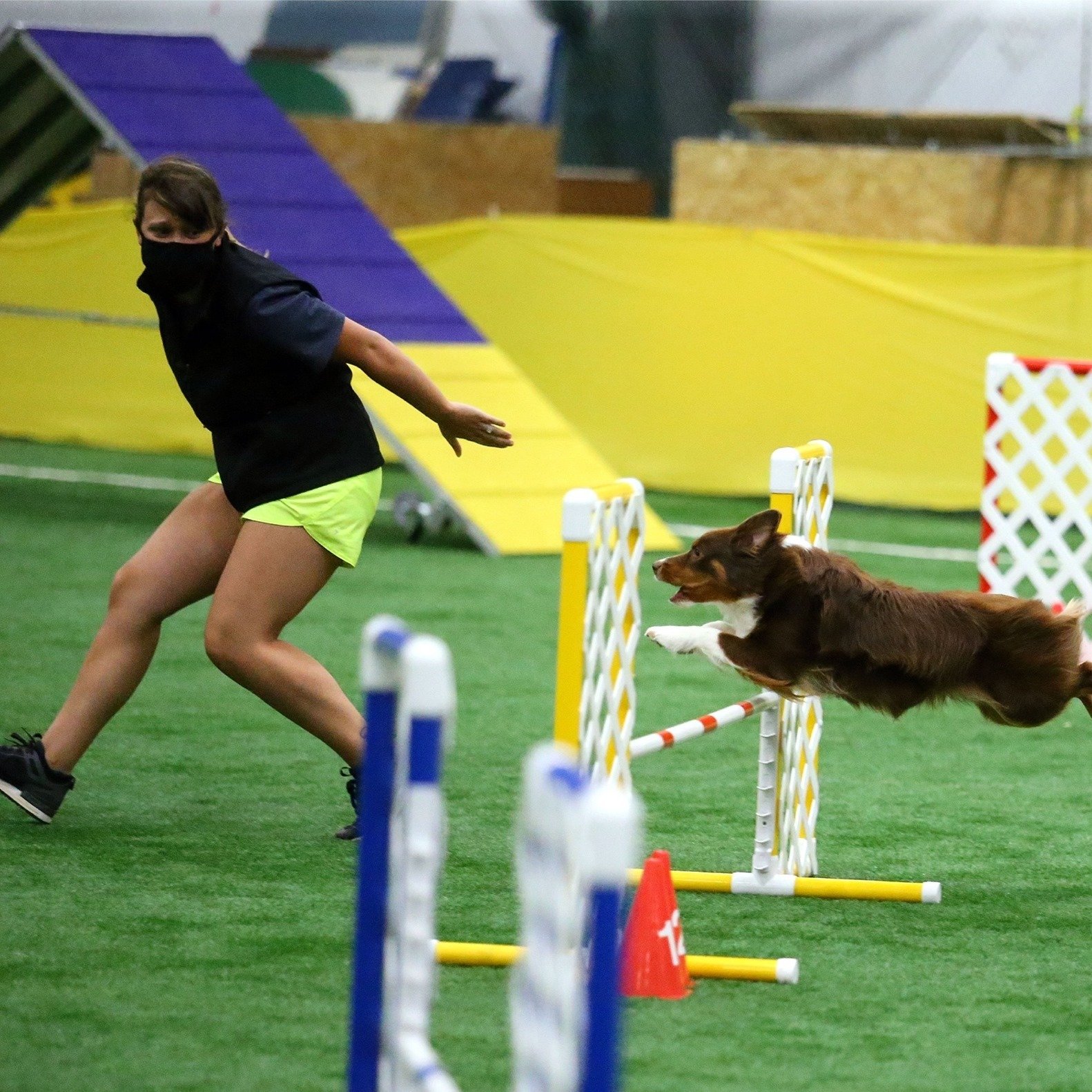In an outdoor setting that appears to be a dog show or training camp, a woman of European descent is seen running alongside a brown and white Cocker Spaniel-like dog that is mid-flight, clearing a hurdle. The woman, who is wearing a black mask, a black shirt paired with a black vest, neon yellow shorts, and black sneakers, is slightly ahead of the dog, seemingly coaching it. The vibrant scene unfolds on green faux grass, and the hurdle, constructed from bright yellow and blue PVC pipes with white lattice sides, stands about three feet off the ground. In the background, other agility equipment, including a yellow and purple seesaw for dogs, can be seen. A decorative yellow banner adds to the festive atmosphere, partially covering some wooden structures in the area.